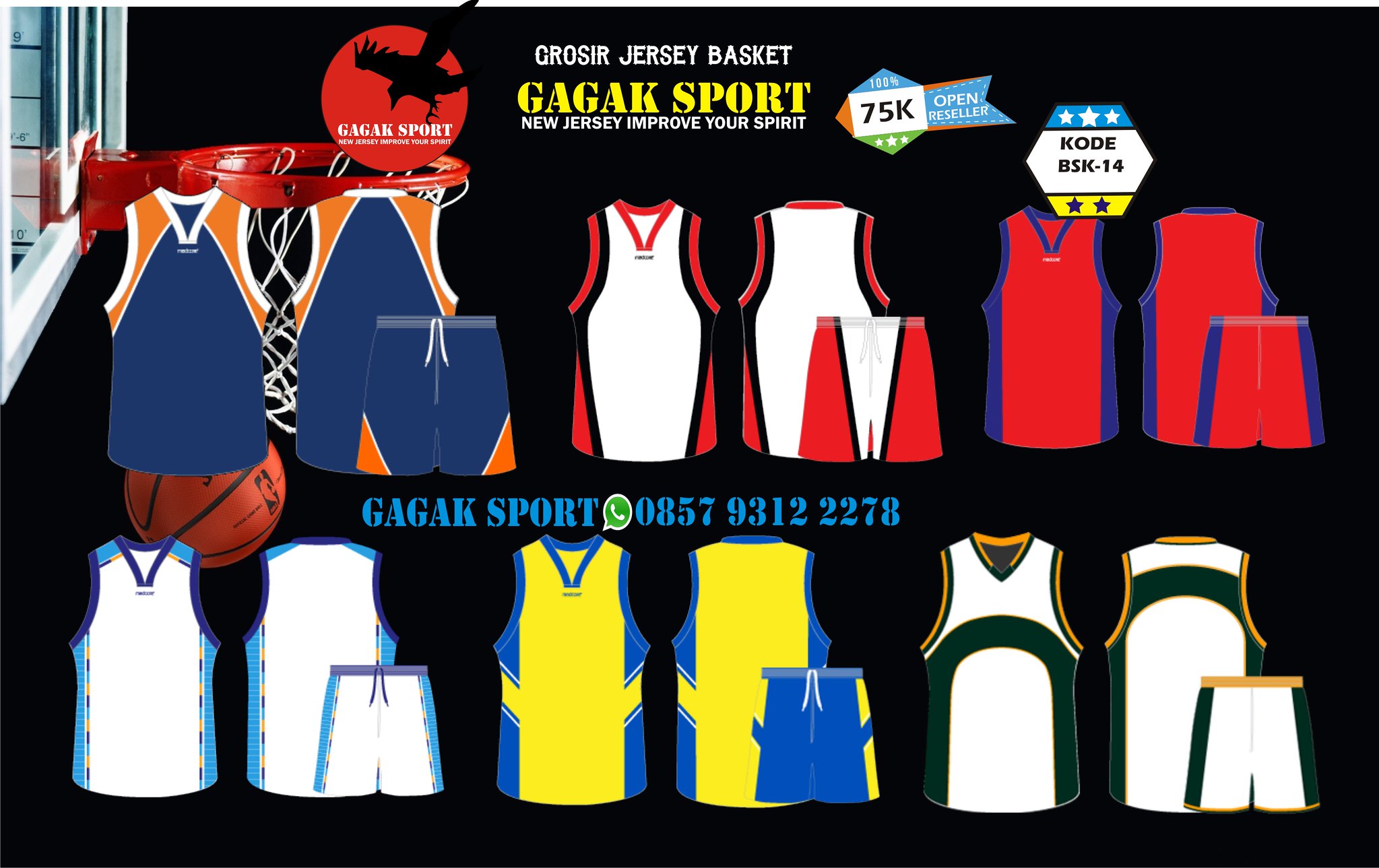This is a detailed graphic advertising basketball uniforms by the company Gag-Guck Sport. The image has a sleek black background and prominently features six sets of basketball uniforms arranged in two rows of three. Each set includes a front and back view of the jersey, along with matching shorts displayed overlapping the back view. The uniforms come in various vibrant color combinations: orange and purple, black, white, and red, red and blue, yellow and blue, gold, green, and white, and light blue, white, and dark blue.

In the upper left-hand corner, a basketball hoop and net are depicted with an orange basketball nearby, adding a dynamic sports element to the design. The company logo is situated prominently within a red circle silhouetted by a black bird, labeled "Gag-Guck Sport." At the top of the image, bold yellow and white text reads "Grossier Jersey Basket, Gag-Guck Sport, New Jersey, Improve Your Spirit," emphasizing the company's New Jersey roots and its motivational tagline. Additionally, there is blue text with a phone number in the middle of the graphic for contact purposes. The entire design exudes a high-energy feel, aiming to attract sporting teams to their high-quality basketball uniforms.